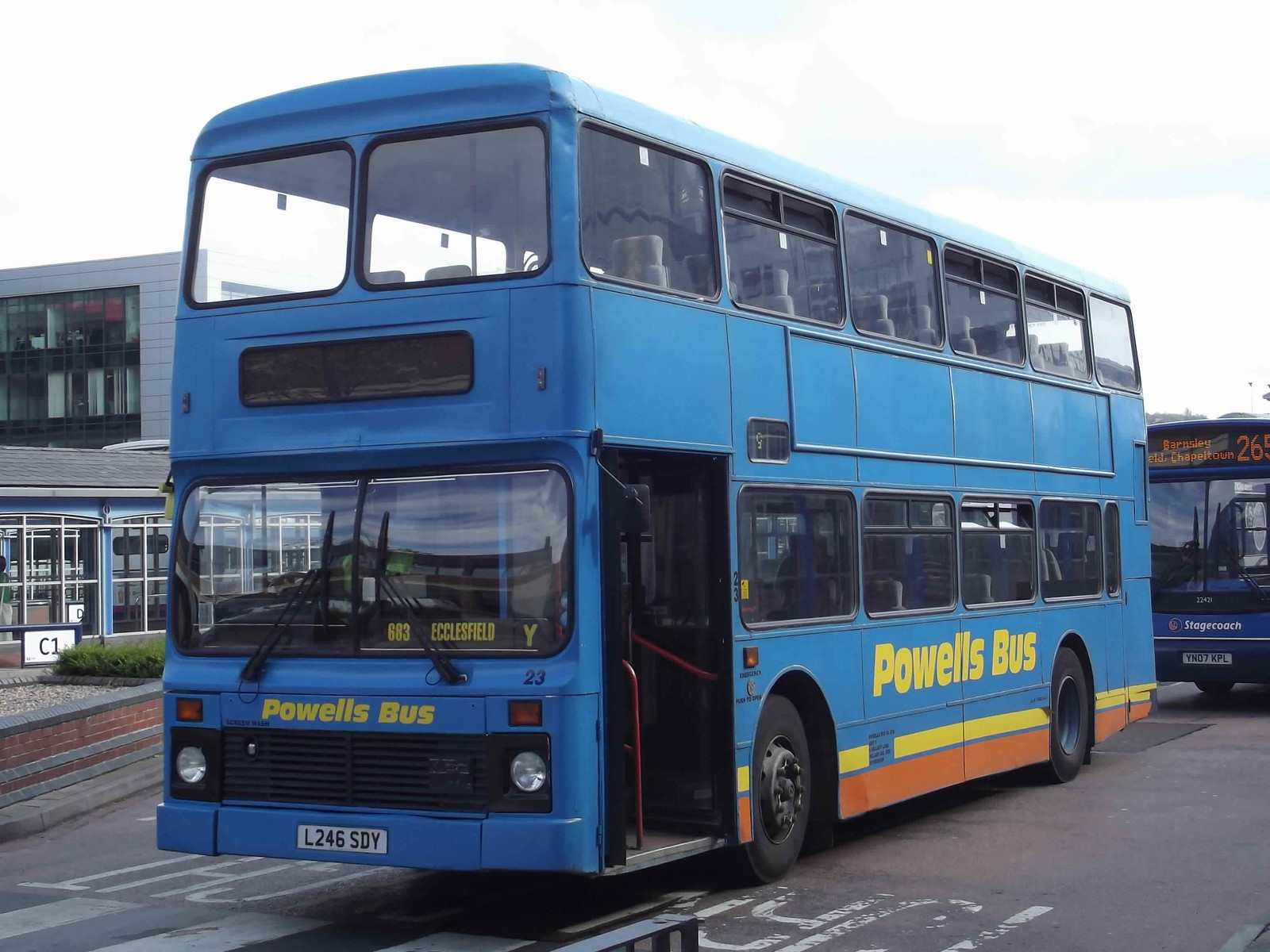The photograph captures a vibrant, blue double-decker bus prominently positioned at the center of the image, parked on a gray asphalt road adorned with multiple white road markings and a distinctive white and gray crosswalk in front of it. This eye-catching bus, bearing the name "POWELL'S BUS" in bold yellow letters on both the front and sides, features distinctive orange and yellow stripes running along its lower edge. In the bus' front window, a sign with yellow text displays the route number "683" and the destination "ECCLESFIELD." The license plate of the bus is marked with the characters "L246SDY."

Adjacent to the Powell's Bus is another bus, a modern, blue public transit vehicle identified as a "Stagecoach." This Stagecoach bus showcases a digital display reading "BARNSLEY CHAPELTOWN 265" and has its license plate labeled "YN07KPL." The setting appears to be urban, with a glimpse of a white brick, two-story building on the left, suggesting that the photo was taken outside, possibly in a bustling part of the city. In addition, the Powell's Bus presents red railings visible through an open door near the front, adding a dash of color contrast to the scene. Despite being stationary, the Powell's Bus exudes a sense of readiness and purpose, captured amidst a typical cityscape.